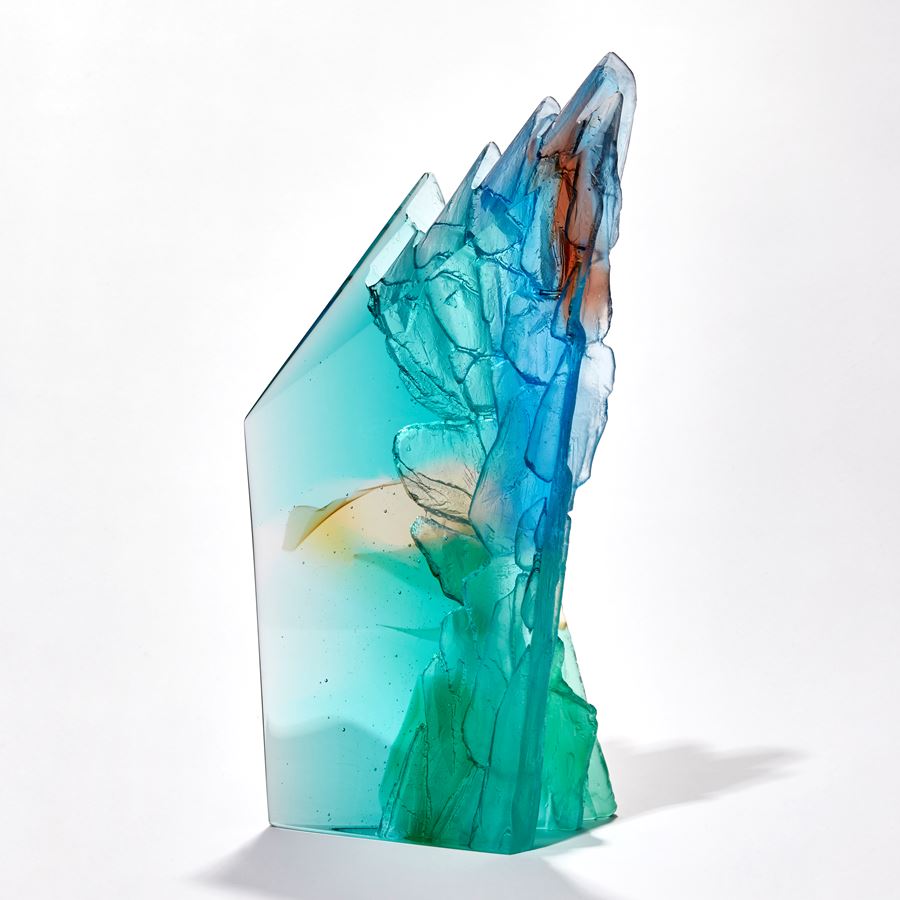The image showcases an abstract artwork against a primarily white, slightly gray background. A shadow beneath the object merges seamlessly with the clean surface it rests on. The piece, which might resemble a crystal or glass sculpture, possesses a multifaceted form. Its base is rectangular and transitions into an intricate, almost mountainous peak with several tips, the highest one pointing towards the upper right of the image.

The artwork features a symphony of colors: the lower section starts with varying shades of green, progresses through a soft marine blue mixed with touches of peach in the middle, and culminates in red hues near the top. The uppermost tip is a blend of blue and white. The front of the sculpture is characterized by a jagged, craggy texture, while the back remains smooth, giving the impression of a carefully crafted, translucent glass collage. The piece is symmetrical, yet its surfaces contrast through a combination of rocky and sleek finishes, creating an engaging visual dynamic. Overall, the statue captures the essence of a fragmented, yet cohesive piece of glass art, echoing both natural and abstract elements.